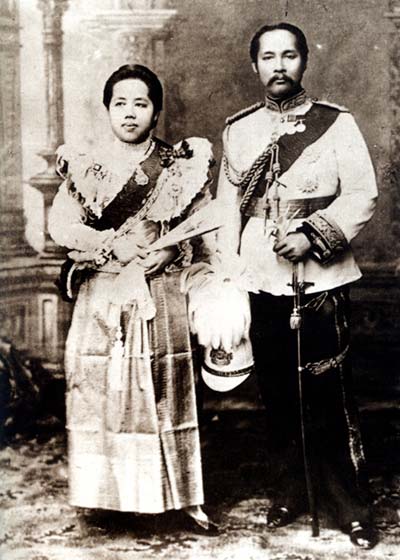The black-and-white historical photograph depicts two oriental figures, a man and a woman, dressed in elaborate traditional attire, posing for the camera. The woman, standing on the left, wears a long, elegant dress adorned with a sash that wraps around her chest and torso. Her outfit includes distinct shoulder pieces, and her dark hair is styled short and possibly tied back. She appears to be holding an object across her midsection, perhaps a fan. 

The man on the right, distinguished by his middle-aged appearance, short black hair, and notable mustache, is dressed in dark shoes, dark pants, and an ornate white military-style uniform. His uniform features intricate embroideries on the neck, shoulders, and cuffs, complemented by a gold belt and a black sash crossing from his right shoulder. He holds a sword pointing downward in his left hand, encased in a black sleeve. Both individuals stand shoulder to shoulder in front of an old-fashioned building or a courtyard, possibly indicating an indoor setting based on the architectural elements. The photo exudes a sense of formality and regality, capturing a moment frozen in time.